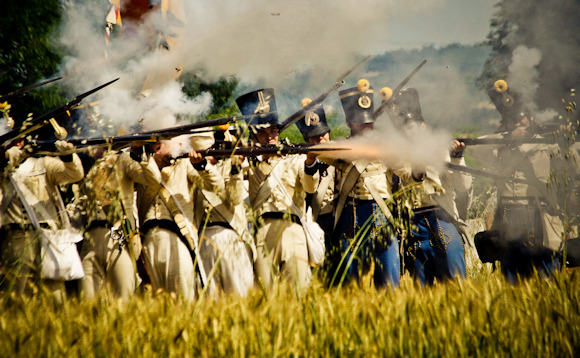In this highly dynamic and smoky scene, a line of soldiers from an 18th-century battle stands poised on a grassy battlefield. The soldiers, primarily clad in white uniforms with dark belts and bayonets affixed to their old-timey, muzzleloading rifles, are captured mid-action as they fire their weapons, sending plumes of smoke and fire into the air. A few of the soldiers in the front wear distinguished blue uniforms complete with tall blue hats adorned with gold pom-poms and matching blue pants. Amidst the white-clad infantry, some soldiers also sport crossed bandoliers slung over their chests. The tall grass of the field reaches just below knee height, creating a setting interspersed with green trees barely visible through the thick, rising smoke. Both the background and the details of a flag behind the soldiers are nearly obscured by the extensive smoke, lending an intense and chaotic atmosphere to the historical battle scene.